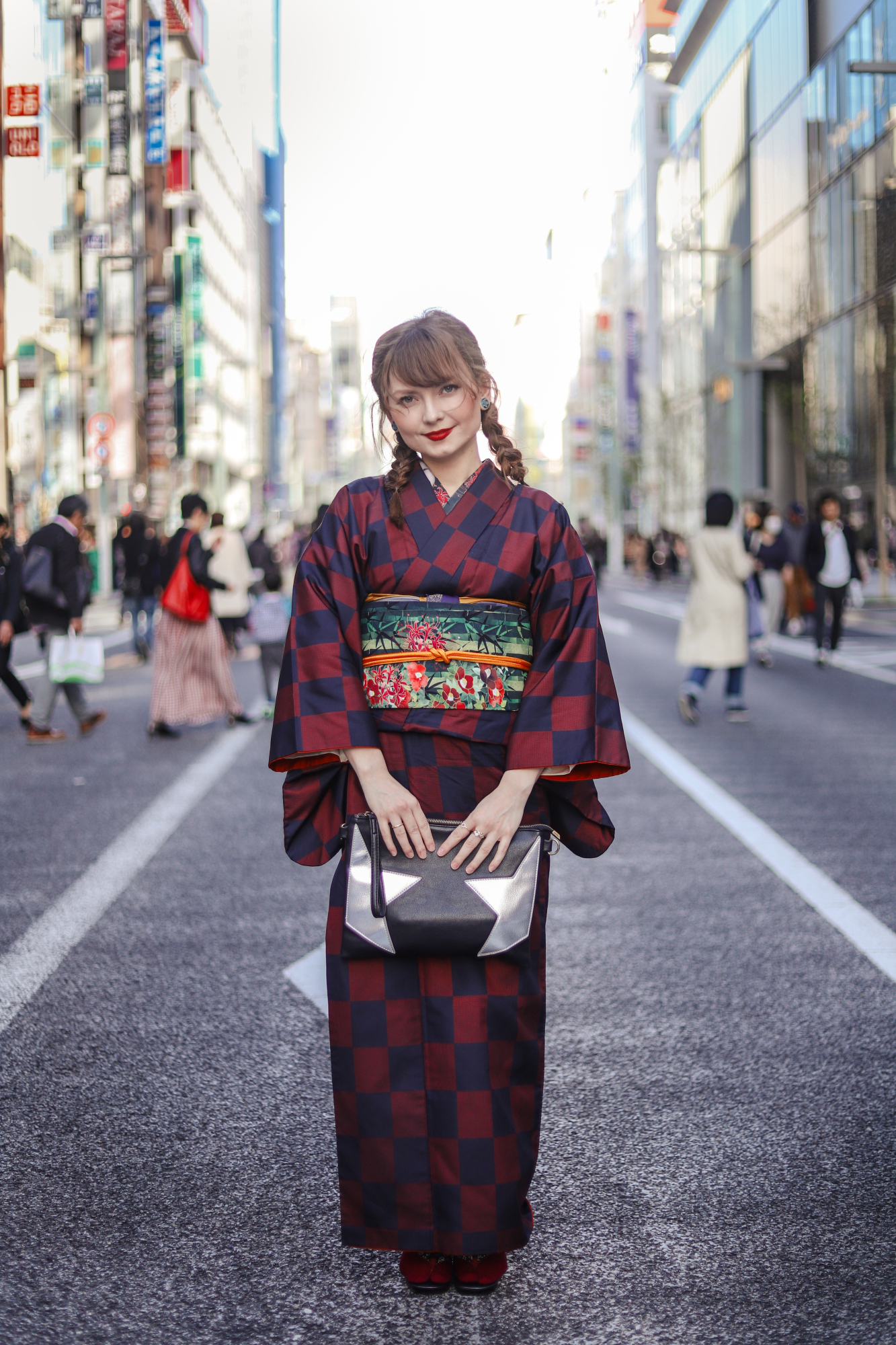A detailed caption for the image could be:

A young Caucasian woman stands confidently in the middle of a busy pedestrian street, likely in Japan, surrounded by tall buildings adorned with Asian characters. She wears a striking black and red checkered kimono, paired with a traditional obi belt featuring green and navy backgrounds with red lotus flowers and orange trimming. Her silvery purse with black leather flaps is clasped in both hands at her waist. Her light brown hair is styled in two pigtails, with one resting over her shoulder and the other cascading down her back. She sports an elegant makeup look, complemented by bright red lipstick and rosy cheeks. Completing her outfit, she wears burgundy-colored flat shoes. The scene is bustling with pedestrians against a backdrop of blurred city life, highlighting the cultural and urban ambiance.